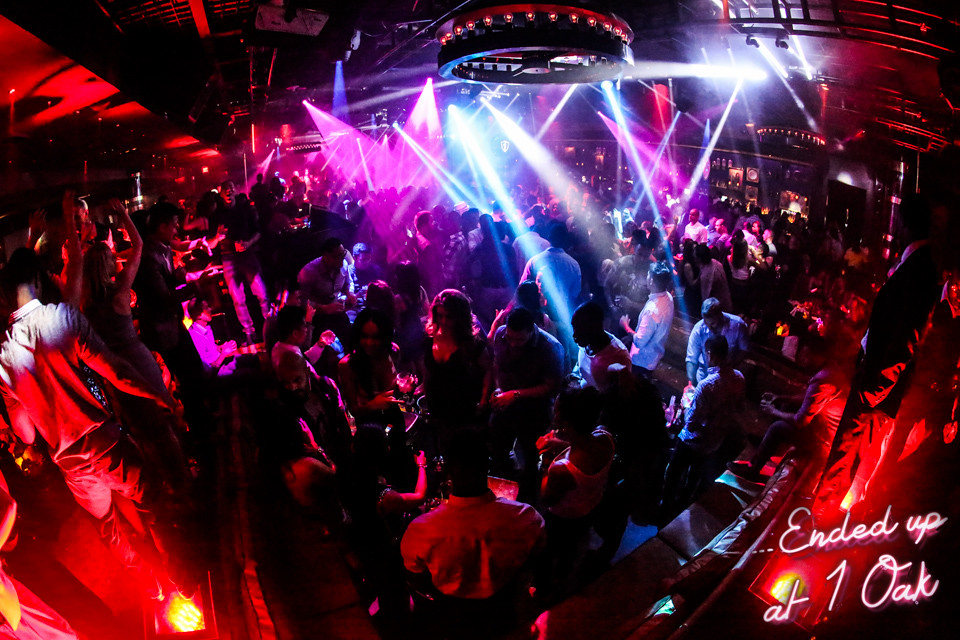The photograph is a horizontal rectangular frame capturing a vibrant scene at the nightclub One Oak in Las Vegas, located at the Mirage Hotel. It appears to be taken from an elevated position, possibly an upper balcony, offering a panoramic view of the dance floor below. The image is bathed in predominantly red, black, neon pink, and blue hues, casting an electrifying ambiance. Spotlights from the ceiling shine down, illuminating various groups of people crowded at the center, either dancing or conversing. Metal frameworks and beams can be discerned along the ceiling, supporting a striking circular red light fixture that resembles a pirate galleon's steering wheel. The club is heavily suffused with neon colors, with streaks of blue and purple light bouncing off the dancers and adding to the dynamic atmosphere. In the lower right-hand corner, written in a cursive white font, is the text "Ended Up at One Oak."